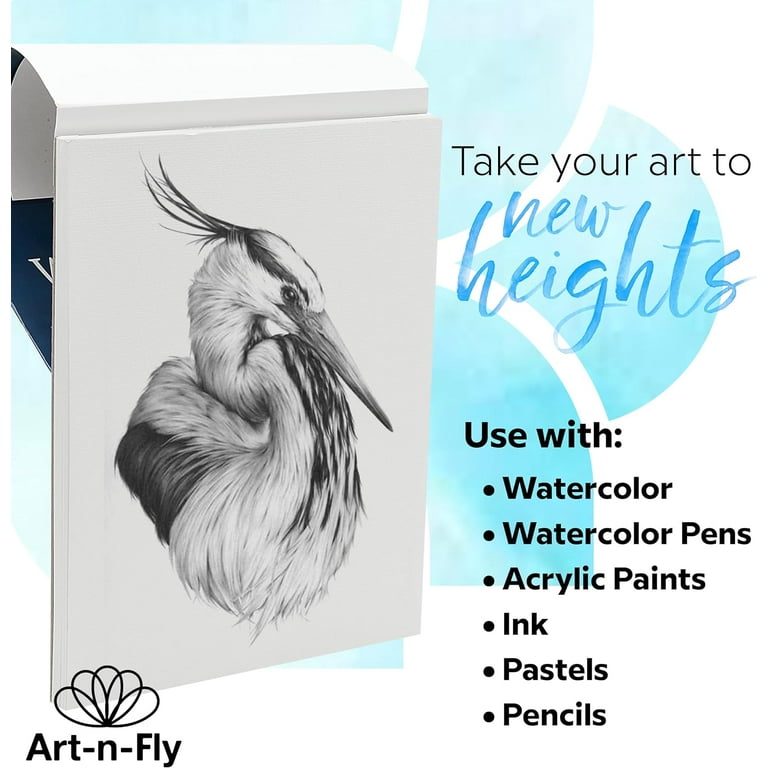This advertisement for Art-N-Fly art paper features a prominently displayed logo of a peacock outline at the bottom left corner. The central focus of the image is a flipped-over sketchbook showcasing a detailed pen and ink drawing of a stork-like bird, primarily shaded in black and white, with intricate dark accents on its body, neck, and beak. Above this sketch, bold black text encourages artists to "Take Your Art to New Heights," with "New Heights" elegantly rendered in a blue calligraphic watercolor style. Adjacent to this motivational message, and following in a bullet-point format, the ad lists the versatile mediums that can be used with the paper: watercolor, watercolor pens, acrylic paints, ink, pastels, and pencils. The background is subtly adorned with light blue semi-circular squiggle designs, adding a touch of creative flair to the composition.